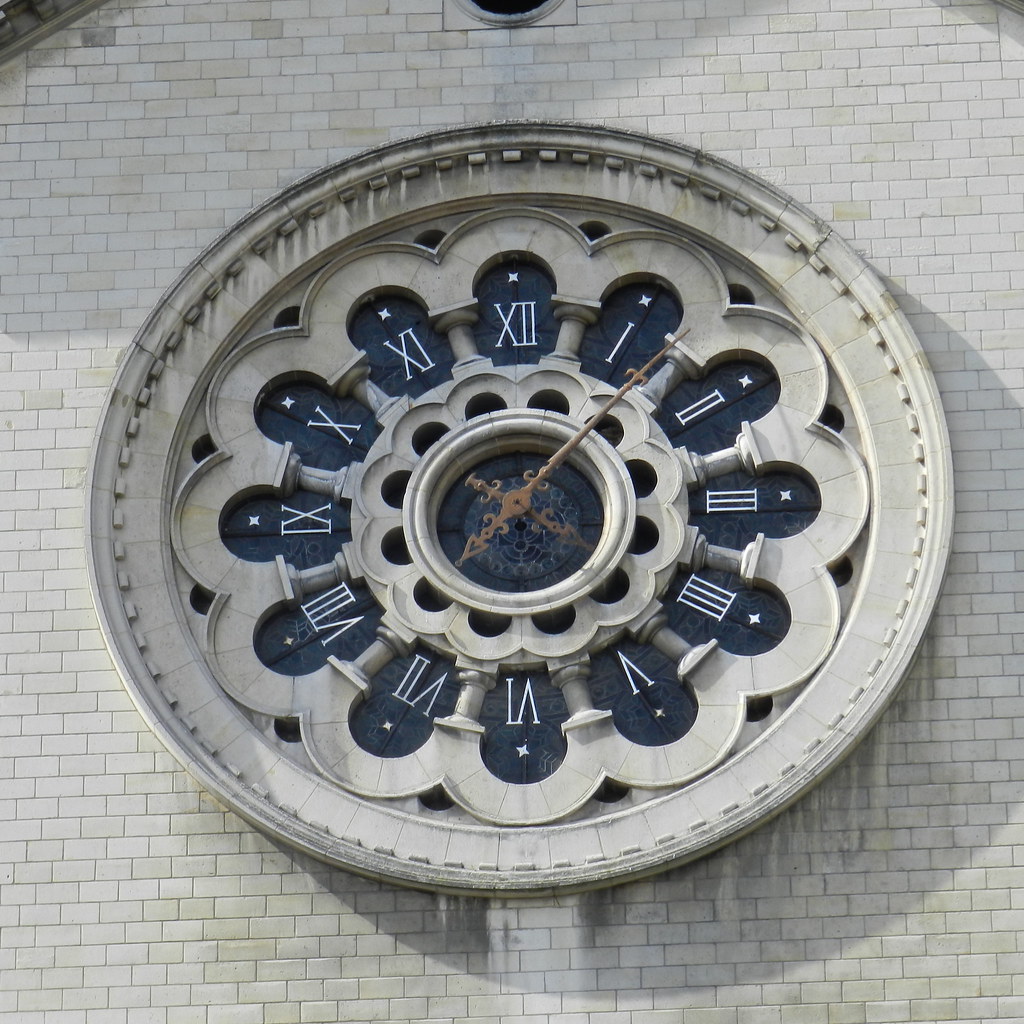This image depicts a close-up view of an oversized stone clock mounted on the white brick façade of a building. The clock, featuring Roman numerals, boasts an intricately designed stone face with subtle blue accents encircling the numerals. Above each numeral is a delicate white star, adding an elegant touch. The top left of the image reveals a slanted structure, likely the building's roof, and the bottom part of another round object emerging from the center top of the picture. Only a partial view of the building is visible, placing the focus squarely on the ornate details of the clock itself.